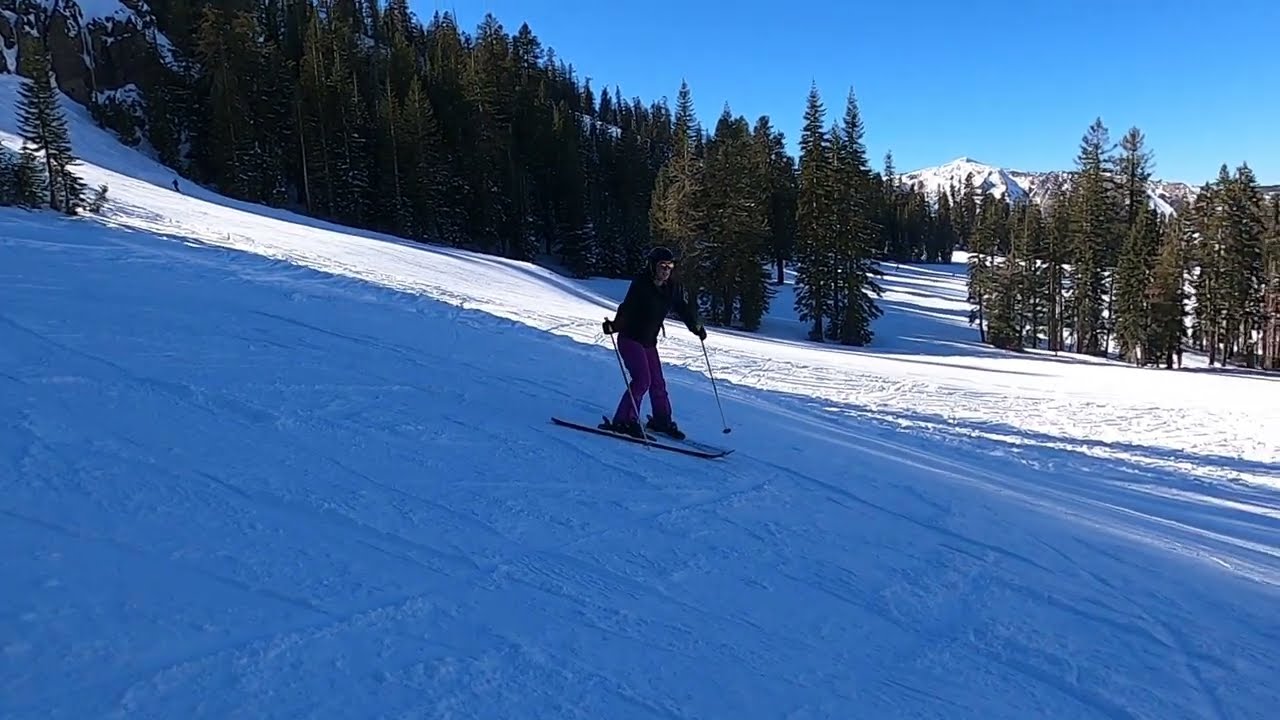This photograph captures a lone skier descending a snowy hill on a bright, clear day with a vivid blue sky. The skier, dressed in a black long-sleeved shirt, a helmet, snow goggles, and magenta-colored pants, is skiing downhill from the upper left to the lower right of the image. They are holding poles in each hand and are positioned in a shadowed area of the slope. The hill has a mild incline with part of it sunlit, creating stark contrasts in the snow's appearance. In the background, there is a dense stand of green pine trees with small openings and their long shadows stretching from left to right, indicating a late afternoon setting. Beyond the trees, a distant snow-covered mountain adds to the scenic backdrop. The entire scene emphasizes the skier's solitary journey and the natural beauty of the snowy landscape.